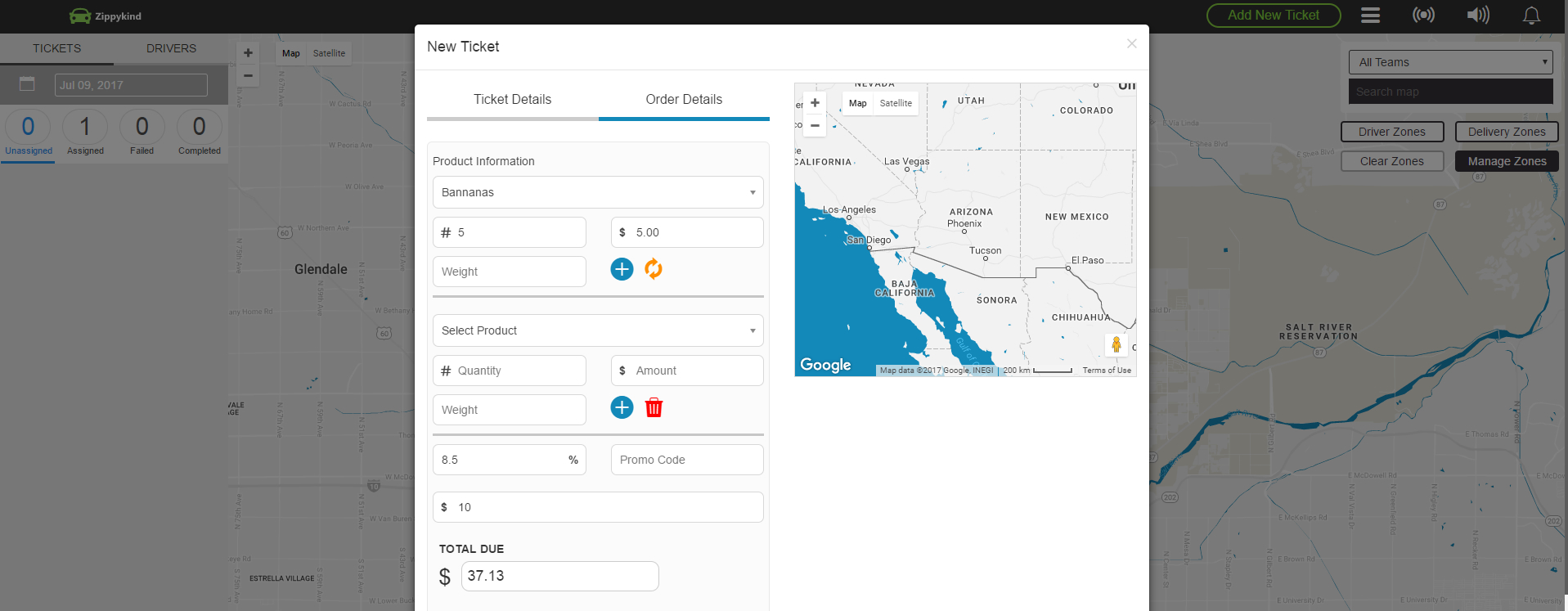This image displays a user interface of a ticketing and product ordering website, rendered primarily in the center of the page. 

At the top of the page, several tabs are visible: "New Ticket," "Ticket Details," "Order Details," and "Product Information." Below these tabs, the website interface is segmented into various input fields and informational boxes. 

The first field displays the word "Bananas" followed by the quantity "5," priced at "$5." Additionally, the term "Wait" is entered within a text box below this line.

Following this is a selection interface containing a dropdown or text box labeled "Select Product." Below this section, there is another text box labeled "Number Quantity," allowing users to specify quantities. A subsequent text box is labeled "Dollar Sign Amount." Another field below this displays the word "Wait."

To the right of these input fields, there is a blue circular button with a plus sign, signifying an option to add items, and next to it, a red trash can icon for deleting entries.

Further down the interface is another text box containing "8.5" followed by a percentage symbol. Below this is a text box labeled "Promo Code" for entering discount codes, followed by another text box displaying "$10."

At the bottom of these fields, the total amount due is displayed as "$37.13" within a text box.

To the right side of this webpage, a Google Map is visible, showing parts of the United States and neighboring regions. The map includes portions of California, Baja California, Nevada, Utah, Colorado, Arizona, and New Mexico, alongside parts of northwestern Mexico, including Sonora and Chihuahua.